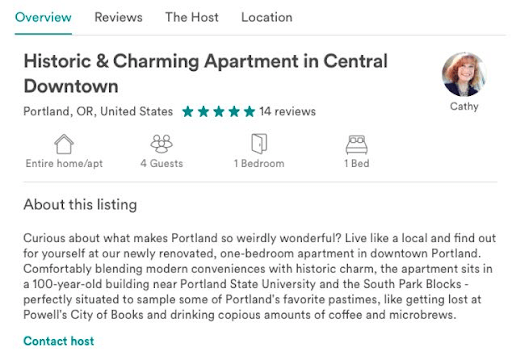**Detailed Caption:**

Screenshot of an Airbnb listing for a historically charming apartment located in Central Downtown Portland, Oregon. The listing showcases high ratings, with a five-star average from 14 reviews. The host, Kathy, who appears in her profile picture as a woman in her mid-30s to 40s, offers an entire home/apartment suitable for four guests. The space includes one bedroom and one bed. 

The overview section highlights the key attributes of the location, emphasizing its blend of modern amenities with historic charm. The apartment is housed in a 100-year-old building near Portland State University, situated in the scenic South Park Blocks. The descriptive text invites guests to explore the quirky and wonderful aspects of Portland, suggesting activities such as visiting Powell's City of Books and indulging in the city’s renowned coffee and microbrews. The listing encourages potential visitors to experience Portland like a local while staying in a newly renovated, comfortable living space.